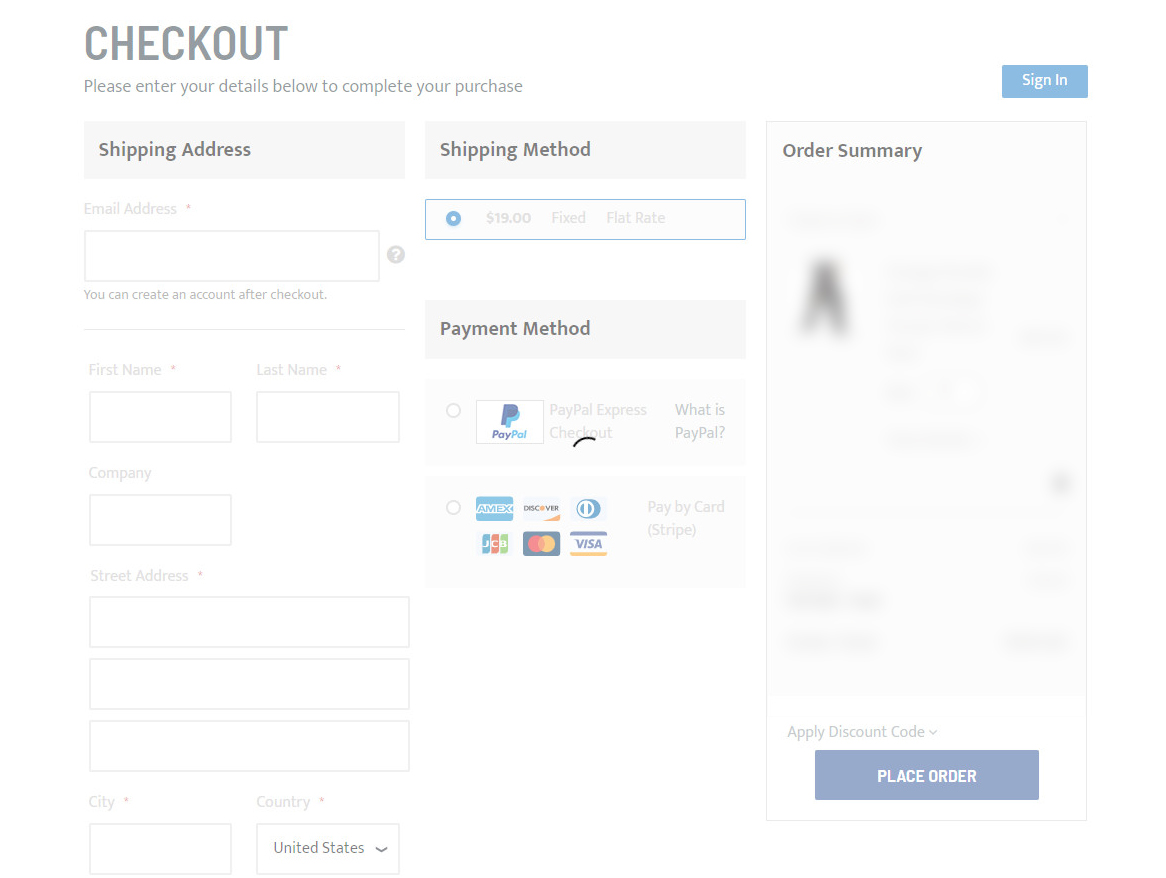This image captures a detailed view of a computer screen displaying a checkout page. At the top, the word "CHECKOUT" is prominently displayed in all gray uppercase letters. Beneath this heading, a prompt reads, "Please enter your details below to complete your purchase."

The page is organized into several sections. First, there is a "Shipping Address" section where users can input their personal information including first name, last name, company, street address, city, and country. The country field is pre-selected to "United States" but includes a drop-down menu for other options.

Next, the "Shipping Method" section showcases a fixed flat rate shipping option priced at $19. This option is highlighted with a blue dot inside a blue-lined rectangle.

The "Email Address" field follows, along with an option to create an account after the checkout process.

The "Payment Method" section allows users to select between PayPal and various credit card options, providing flexibility for their preferred payment choice.

On the right side, there is a blue "Sign In" button for returning users. Directly beneath this button is an "Order Summary," which has been blurred out for privacy reasons.

Finally, at the bottom of the page, users are given the option to apply a discount code before finalizing their transaction with a blue "Place Order" button.